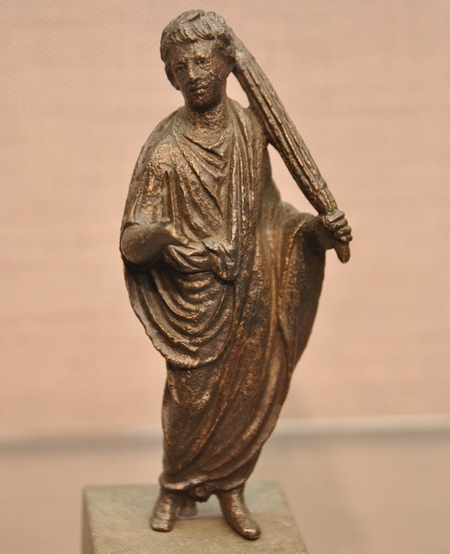This image features a small, aged statue of a man, potentially from the Greek or Roman period, standing atop a square pedestal. The statue, which appears to be made of a deteriorated copper or bronze, exhibits an intricate, rusted, orangish-brown hue. The man, adorned in flowing, toga-like robes and shoes, has a full head of hair. His left hand holds what appears to be a long club or weapon, possibly resembling a sword in a sheath or a ridged walking stick, which rests against his shoulder and extends slightly past his head. His right hand is extended forward, as if reaching out or trying to attract attention. The background features a hard floor and a light peach-colored wall, possibly with a red-pink tint or a brick-like appearance. The statue is positioned slightly off-center, with its gaze directed towards the left side of the image.